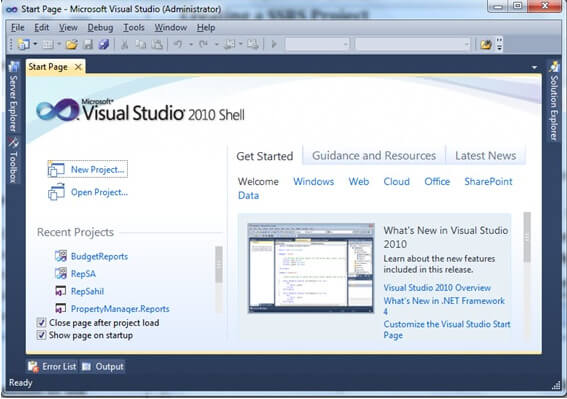Screenshot of Microsoft Visual Studio 2010 Shell Administrator Interface:
This screenshot captures the user interface of the Microsoft Visual Studio 2010 Shell, showcasing an older system with several distinct sections and functionalities. The top menu bar displays options such as File, Edit, View, Debug, Tools, Window, Help, and Start Page. The interface also includes tabs labeled 'Get Started,' 'Guidance,' 'Resources,' and 'Latest News.'

The main window of the program is divided into several columns and boxes, likely representing various tools and data being managed within the program. Toward the lower half of the screen, there are checkboxes labeled 'Budget Reports,' 'Scrap,' 'Close Page After Project Load,' 'Show Page on Startup,' 'Error List,' 'Output,' and 'Ready.'

Additionally, a sidebar or secondary window offers guidance on new features and updates, helping users to stay informed about the latest enhancements in Visual Studio 2010. The overall layout and design reflect the typical interface style of early 2010s software development tools.